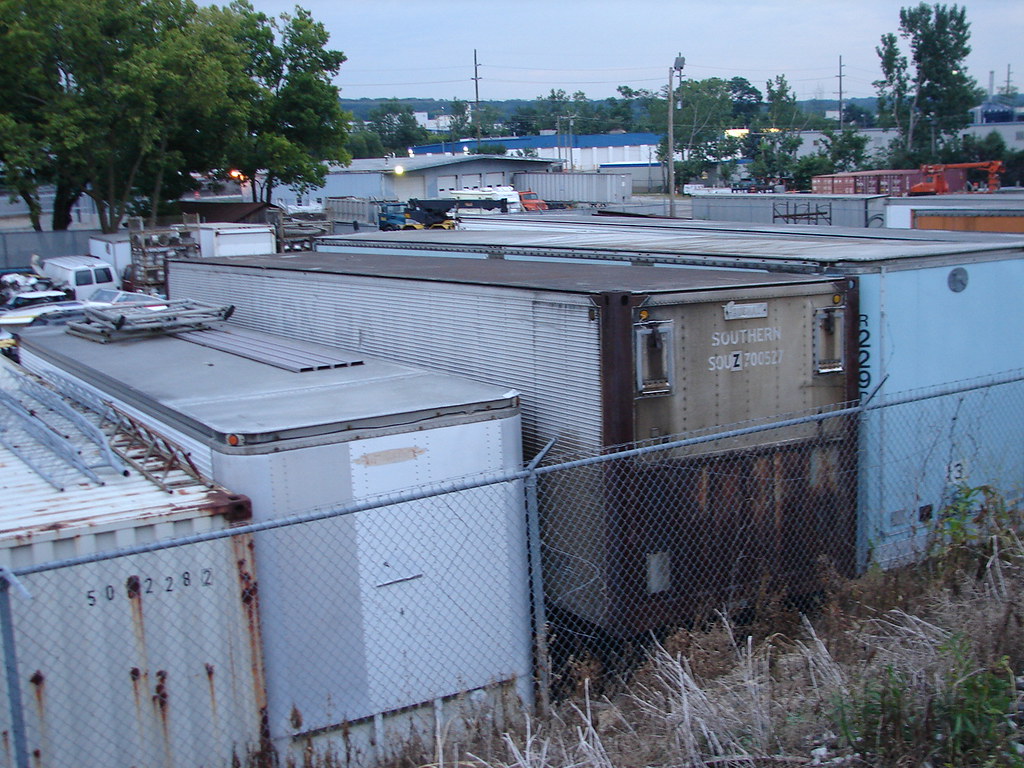The photograph captures an outdoor industrial scene from an elevated perspective. In the bottom right-hand corner, green grass and leaves are visible, alongside branches and twigs in shades of beige and brown. A sturdy chain-link fence, about 8 to 10 feet tall with barbed wire at the top, encloses the area, ensuring security. The fence features square openings that allow visibility through to the inside, where numerous semi-trailers are parked in a row against the barrier.

The semi-trailers vary in appearance: on the left, a white trailer with rust and dirt marks, identified with the numbers "502282"; beside it, a larger white and gray trailer; then a brown and silver trailer bearing the number "32"; followed by a trailer with a silver top and blue sides displaying "R229". The back of one brown trailer also has the word "Southern" written on it. In front of the trailers, several vans and trucks are lined up, including a notable white van.

Further into the background, a gray and white warehouse is discernible, with one semi-trailer backing into its loading dock. Adjacent to the warehouse is an orange crane, surrounded by storage containers. Additionally, the horizon reveals the outline of a cityscape, providing context to the industrial foreground. Green trees dot the scene, adding a touch of nature to the otherwise industrial landscape.